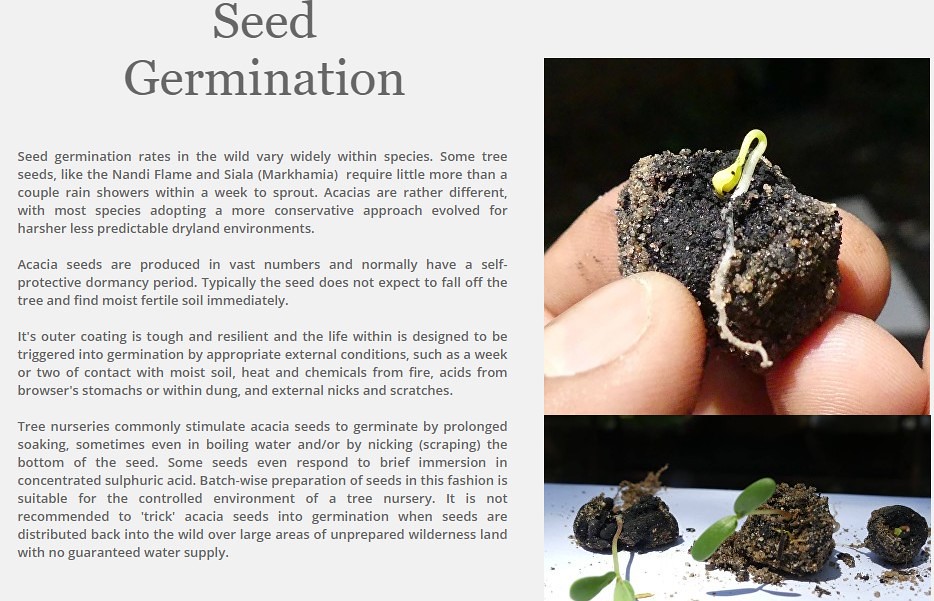The image features a white background with the title "Seed Germination" in large, centered black text (with a capital "S" and "G") on the left side. Below the title are four detailed paragraphs explaining the variability of seed germination rates in the wild. It mentions that species like Nandi Flame and Siala Markhamia can sprout with just a few rain showers, while Acacias require a more conservative approach due to their adaptation to harsher, less predictable dryland environments. The paragraphs further describe the characteristics of acacia seeds, including their dormancy period and stimulation methods like prolonged soaking or boiling water used in tree nurseries. On the right-hand side, the image displays a close-up of someone's hand holding a small sprout embedded in soil. Beneath this, there is another picture showing multiple clumps of soil with sprouts lying on a table, some beginning to poke up and grow leaves.